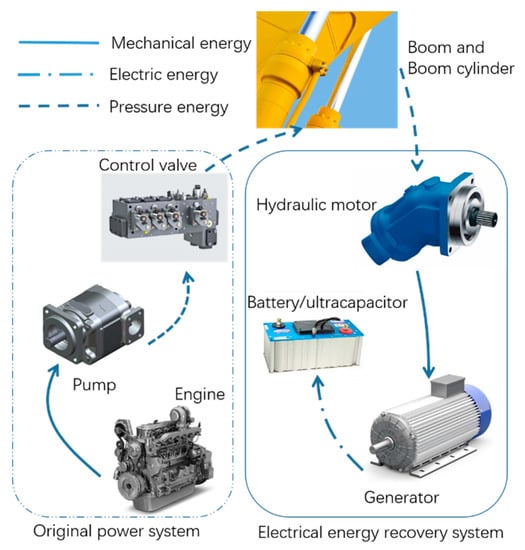The image is a detailed informational graph that visually explains the workings of two different power systems—mechanical and electrical—using varied imagery and a line chart. The chart uses a solid blue line to represent mechanical energy, a blue line with dots to signify electric energy, and a dotted blue line for pressure energy. On the right side of the diagram, an arrow from a dotted blue line leads to a blue hydraulic motor. Nearby, a solid blue line directs attention towards a generator, and a blue and dotted blue line points towards both a battery and an ultra-capacitor. The top right corner depicts a crane component labeled as "boom and boom cylinder."

On the left side, the diagram features an engine connected by a solid blue line to a pump, which then links via a dotted blue line to a control valve. The elements within the image bear labels such as control valve, hydraulic motor, battery, ultra capacitor, pump, engine, generator, mechanical energy, electric energy, and pressure energy. The depicted colors include silver, gray, black, yellow, blue, and red, further demarcating the components of the original power system and the electrical energy recovery system.